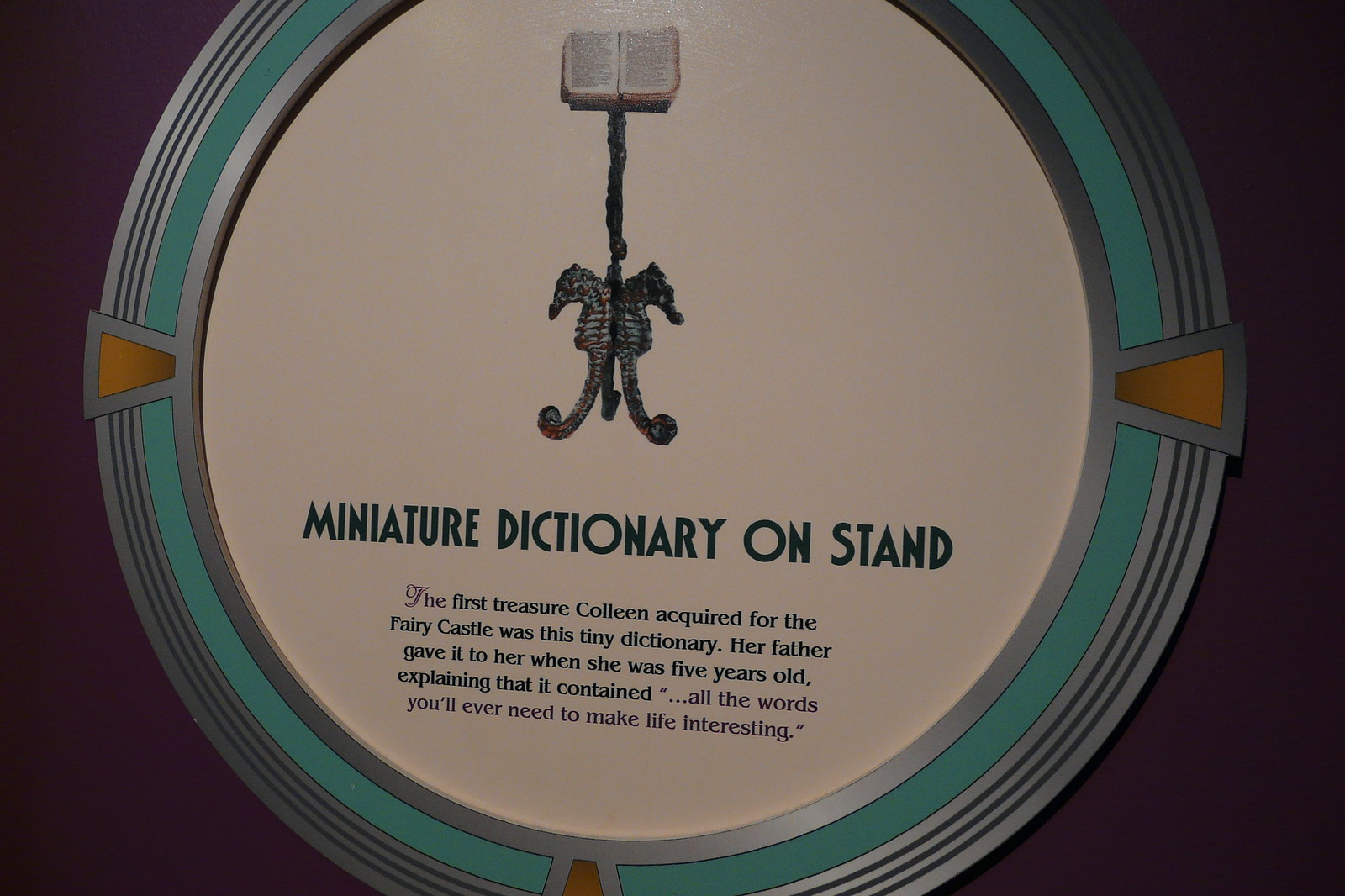The display at the museum features a fascinating circular exhibit set against a purple background. The outer circle is ringed with silver, featuring three bluish lines followed by a turquoise circle, another silver line, and an outlined gold triangle at three points. At the center, the main focus is a miniature dictionary supported by an elegant stand. The intricate base of the stand, consisting of three seahorses facing different directions, supports a vertical bar that holds up the tiny book. The dictionary’s pages are filled with small, black text on white paper, but the content is too tiny to make out. Below this central image, a caption reads: "Miniature Dictionary on Stand." It further explains, "The first treasure Colleen acquired for the fairy castle was this tiny dictionary. Her father gave it to her when she was five years old, explaining that it contained all the words you'll ever need to make life interesting." The text is predominantly in black, with certain emphasized words in gray.